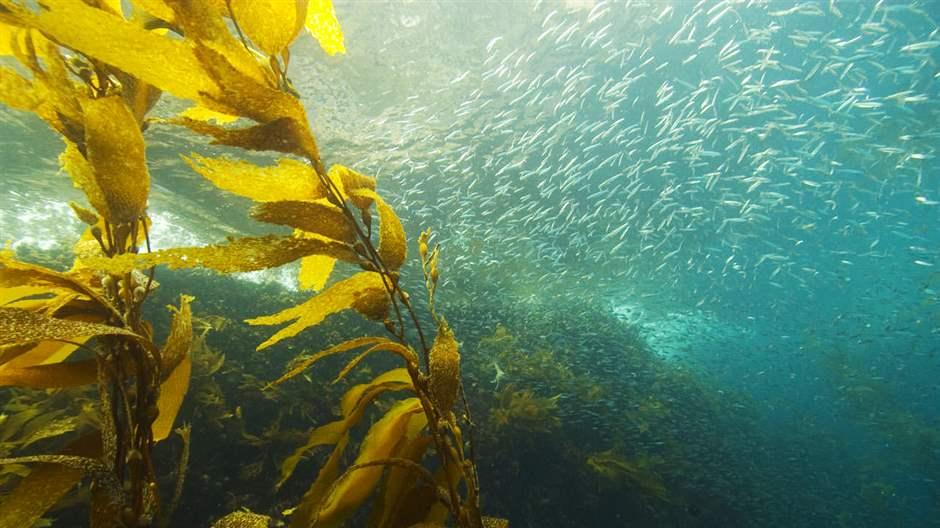The image captures a vibrant underwater scene in the deep ocean, bathed in strong sunlight from above. The water is a mix of blue and green hues, and you can see a dense school of slender, silvery fish—possibly sardines—taking up most of the photograph, creating a shimmering silver cloud that's difficult to see through. In the foreground, two prominent stalks of golden-yellow seaweed stand out, their leaves waving gently. Below and to the left, a dark mound or rock formation adds texture to the ocean floor. In the background, the faint outline of a coral reef can be discerned amidst the schooling fish, and a patch of cream-colored light illuminates the left upper quadrant of the image.